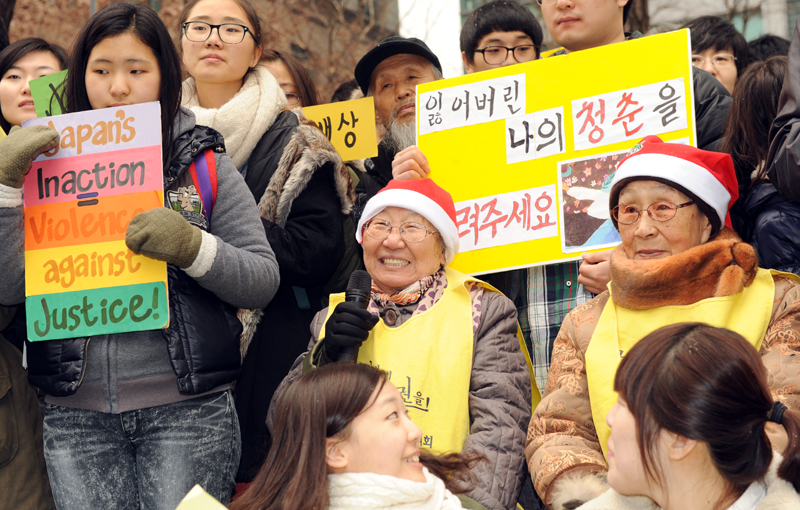In this horizontally aligned rectangular photograph, taken during Christmas time, we see a diverse group of Asian individuals gathered outdoors, likely participating in a peaceful protest or rally. Many of the people, ranging in age from their 20s to their 80s, are adorned in festive Santa hats with white borders and red tops, adding a holiday touch to the scene. Several individuals, especially the two older women in the foreground, are smiling and appear relaxed. These women are also wearing yellow vests over their coats, which display black symbols, and have wire-rimmed glasses. 

Central to the image is an older lady holding a microphone, possibly delivering a speech. In the background, multiple signs are visible. One sign, held by a person standing behind the two elderly women, features a yellow background with various paper cut-outs bearing black or red symbols. Another prominent sign, carried by a younger woman in the left side of the photograph, reads "Japan's inaction violence against justice," with each word written on different colored backgrounds and in various colored markers. Some signs have Japanese characters, indicating a blend of languages used to convey their message. The participants' peaceful demeanor contrasts with the serious message displayed on their signs, suggesting a call for justice rather than a display of violence.